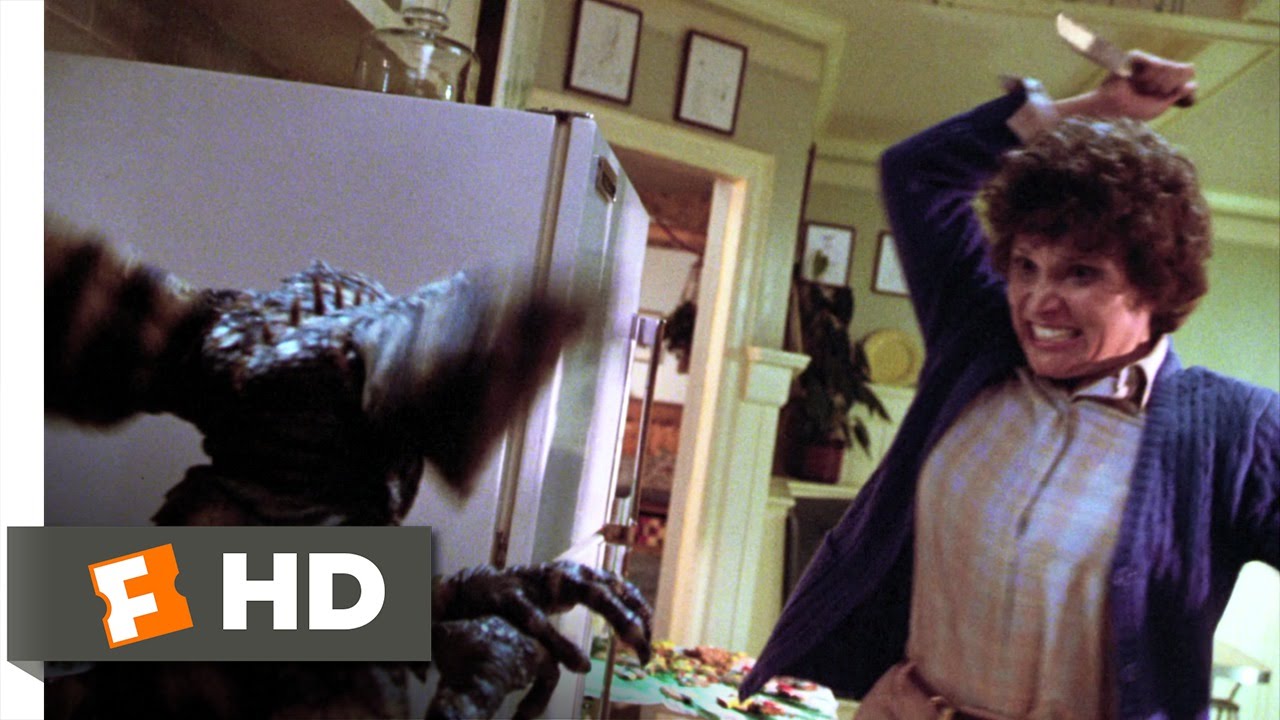This detailed movie still image, potentially from the 1980s film "Gremlins," features a tense scene set in a kitchen. The focal point on the right side is a woman with short, curly hair, dressed in a blue sweater over a white and yellow collared shirt and light pants. She holds a knife in her right hand, raised high as if about to strike, her face fierce with determination and mouth open in a snarl. Opposite her, on the left side of the image, is a foreboding gremlin creature seen from behind, with large bat-like ears and long claws, its reptilian, almost alien form casting a menacing presence. The background includes a white fridge and framed images on the wall, emphasizing the kitchen setting. The image has a gray banner in the bottom left corner with the Fandango logo, showing a stylized orange movie ticket with a white 'F,' and the letters "HD" and "FHD." The overall aesthetic and details suggest the scene dates back to the 80s, enhancing the retro horror ambiance.